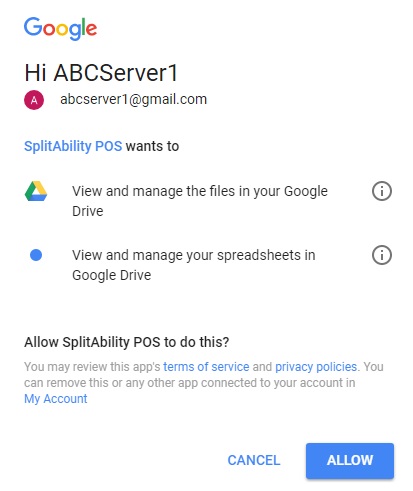The image shows a screenshot from a phone displaying a Google authorization request page. The screen has a clean, white background without any information about time, battery life, or notifications at the top. 

At the very top of the screen, the classic multicolor Google logo is prominently displayed, featuring the familiar blue, red, yellow, blue, green, and red letters. Directly beneath the logo, the text "HI" is written in a bold, black font, followed by "ABCS" in all capital letters. Below it, the phrase "ABC server 1" appears, indicating the name of the server.

Further down, there is a red icon with a white 'A' in the center. Adjacent to this icon, the text "ABC server 1 at gmail.com" is written in lowercase letters. Following this, the term "SplitAbility" is presented with the 'S' and 'A' capitalized, and then the acronym "POS" in all capital blue letters.

The next section outlines permissions being requested: 
1. The Google Drive icon is listed with the ability to "view and manage files in your Google Drive" alongside an available information button.
2. A blue dot indicates the option to "view and manage your spreadsheets in Google Drive," also accompanied by an information button.

At the bottom, the text prompts the user to "Allow SplitAbility POS to do this?" Users are given the choice between "Cancel" or "Allow" via buttons at the bottom of the screen, with the "Allow" button featuring blue background and white lettering.